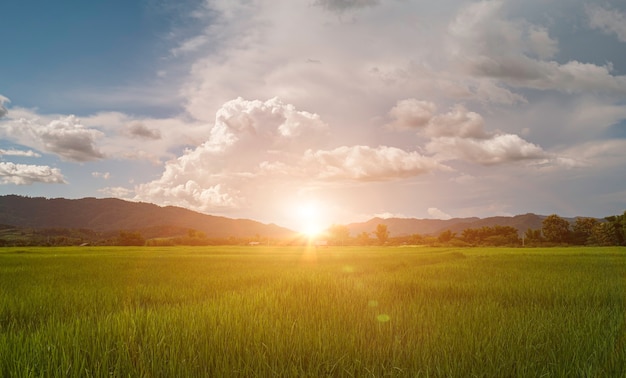In this detailed landscape photograph, a serene grassy field extends across the foreground, where tall, vibrant green grass sways gently, suggesting the frequent passage of wildlife through the area. The field stretches out towards a distant horizon lined with scattered deciduous trees and bushes. Beyond this vegetative boundary, a range of low-lying mountains rises, their peaks bathed in the warm, diffused light of a setting sun, creating an almost mystical ambiance as the sun appears to nestle into the mountain peaks on the left. The sky above transitions from a darker aquamarine blue to clearer hues as one looks upwards, punctuated by a blend of wispy and fluffy clouds that grow thinner and sparser away from the horizon, allowing glimpses of the deepening blue sky. The interplay of light and shadow evokes a photorealistic quality, making the image both captivating and tranquil.